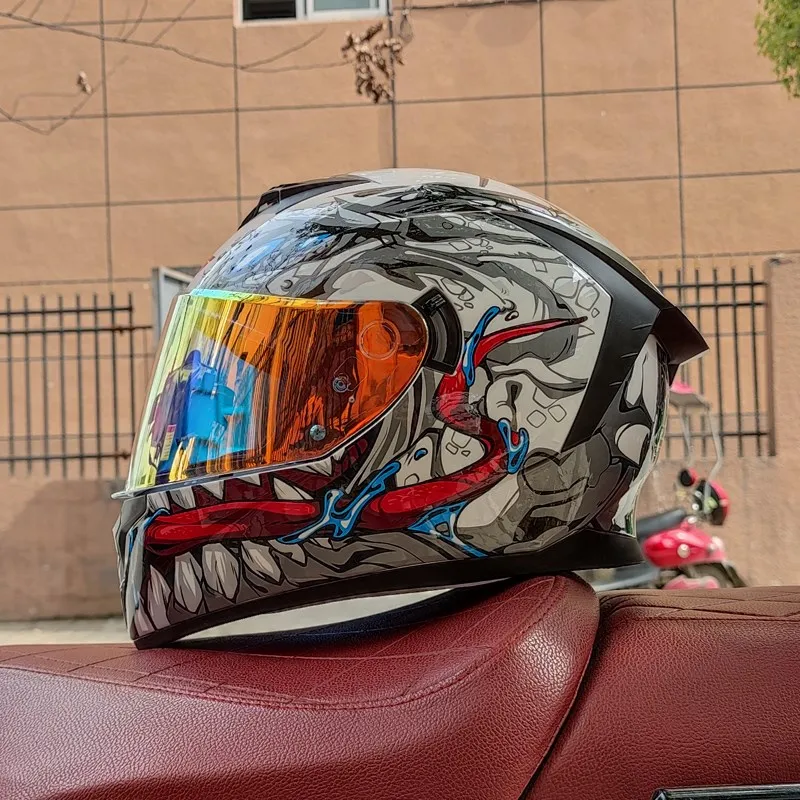This is a detailed photograph of an elaborate motorcycle helmet resting on a motorcycle with a wine red leather seat, featuring intricate stitching. The helmet dominates the frame with its striking design. It has a black and gray background adorned with a vivid, multi-colored visor that reflects hues of blue and amber. The artwork on the helmet depicts a sinister mouth with sharp, gray teeth highlighted in white and a protruding red tongue, giving it a demonic, skull-like appearance. The image is set outdoors on a city street, where a tan brick building with a wrought iron-topped fence forms the backdrop. Additionally, in the background, a small vehicle or bicycle is parked just behind the motorcycle, contributing to the urban setting.